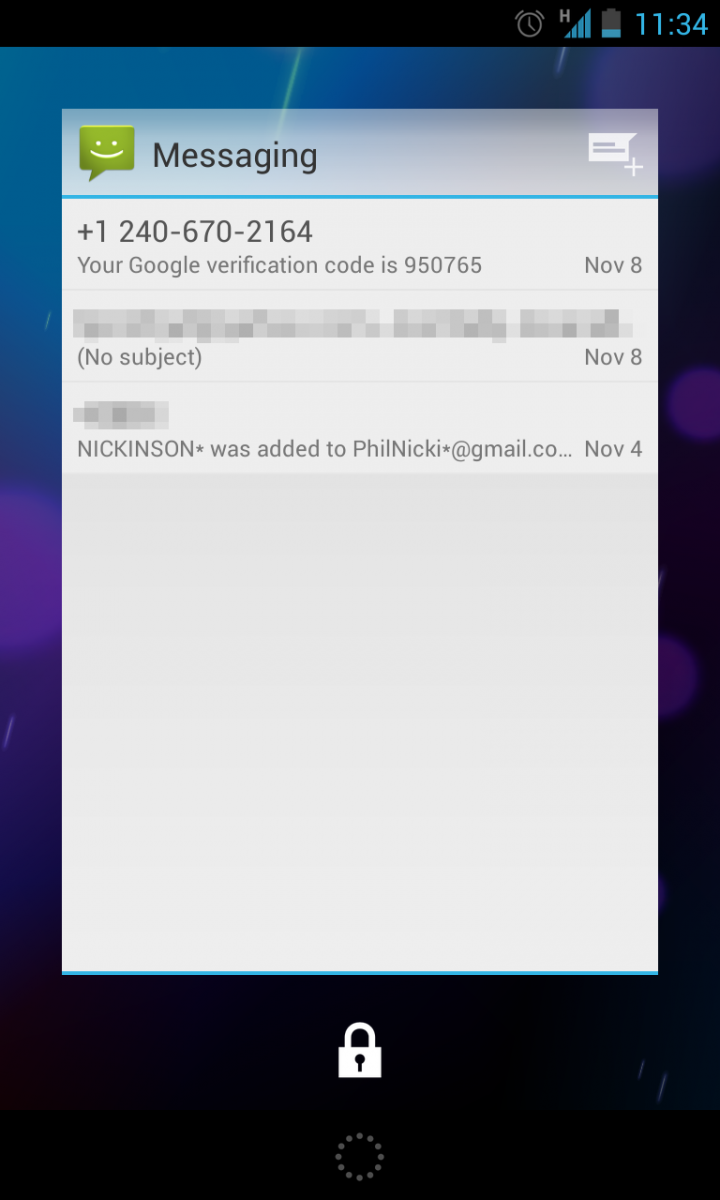A detailed caption for the described image could be:

"A phone screenshot captured at 11:34 shows a message from the number +1 (240) 670-2164. The message contains a Google verification code '950765' dated November 8th. The subject line is blurred out and is marked as "(no subject)". Additionally, there is another blurred line above a message stating 'Nickitsin was added to philnickiasteroid@gmail.com' dated November 4th. At the bottom of the screenshot, a locked icon is visible, with a circular navigation icon indicative of standard smartphone interface elements."